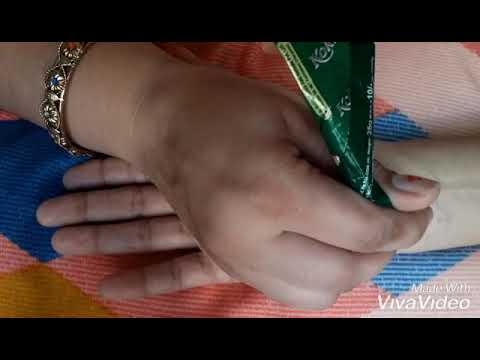The image depicts two hands. The right hand is lying palm up, with the wrist on the right side and the fingers on the left, displaying four visible fingers. This hand rests on a fabric surface patterned with blue, pink, and light pink cubes. The left hand, emerging from the upper left, holds a green item under its thumb and between its index finger. This item, described as twisted green paper, has gold-colored text displaying the letters "KO". The left hand, which appears to be thicker and of a brown-skinned female, wears a gold-colored bracelet adorned with blue and red gems. The scene is bordered by long, horizontal black bars at the top and bottom. In the bottom right corner, white text reads "Made with Viva Video".